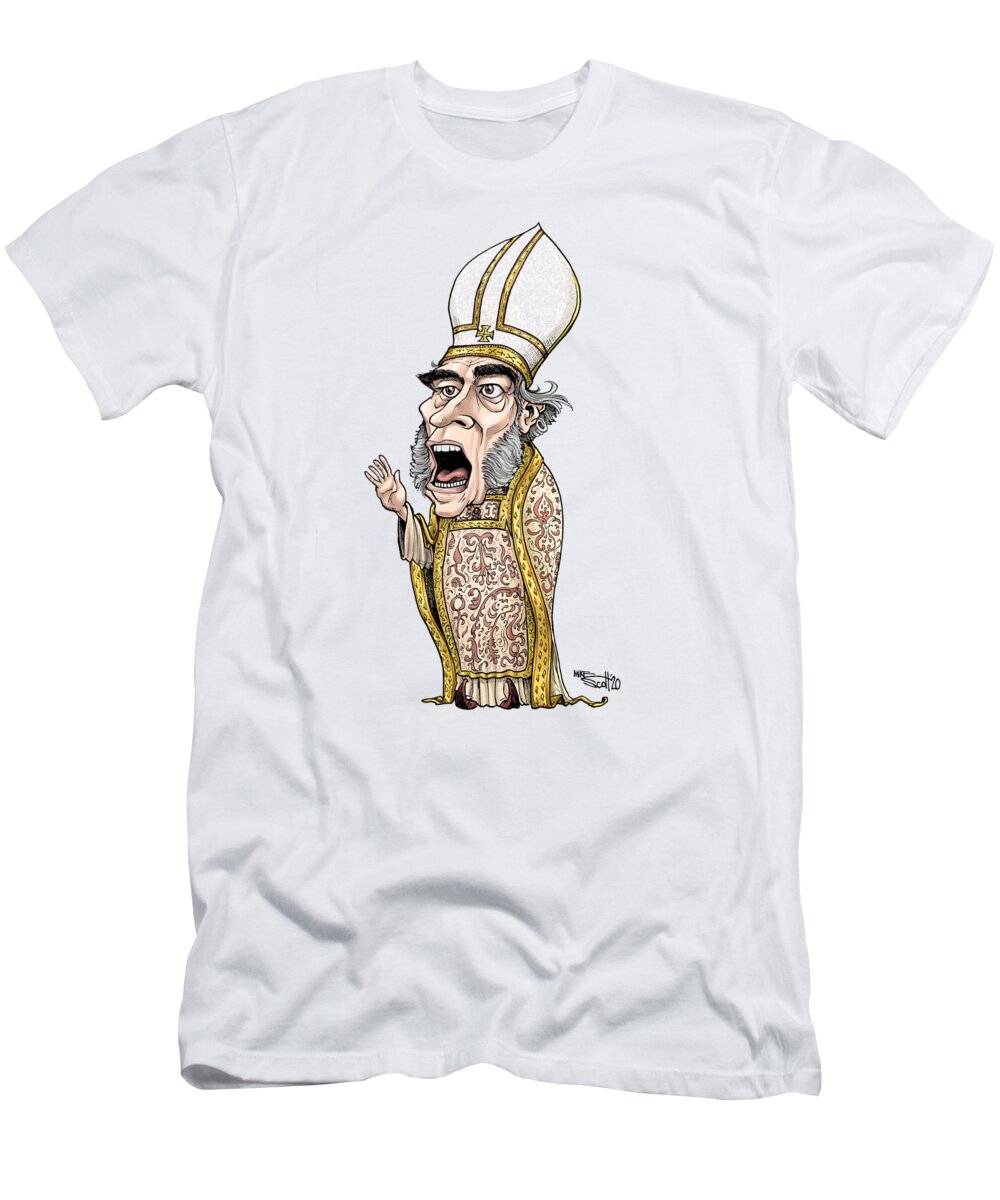This is a detailed color photograph of a short-sleeved, crewneck white t-shirt, set against a plain white background. The t-shirt features a vibrant screen-printed image at the center, depicting a cartoonish clergyman, likely inspired by a Catholic or Orthodox priest. The priest character, who has exaggerated features with large gray sideburns, long gray hair, and prominent black eyebrows, wears a white, pointy hat adorned with gold trim. His mouth is wide open, revealing a pink tongue and teeth, suggesting he is saying something animatedly. His right hand is raised in the air. He is dressed in an elaborate white and red robe also trimmed with gold, and at the bottom, he appears to be wearing red shoes beneath a pleated skirt-like garment. A black signature is visible below the graphic, adding an artist's touch to the design.